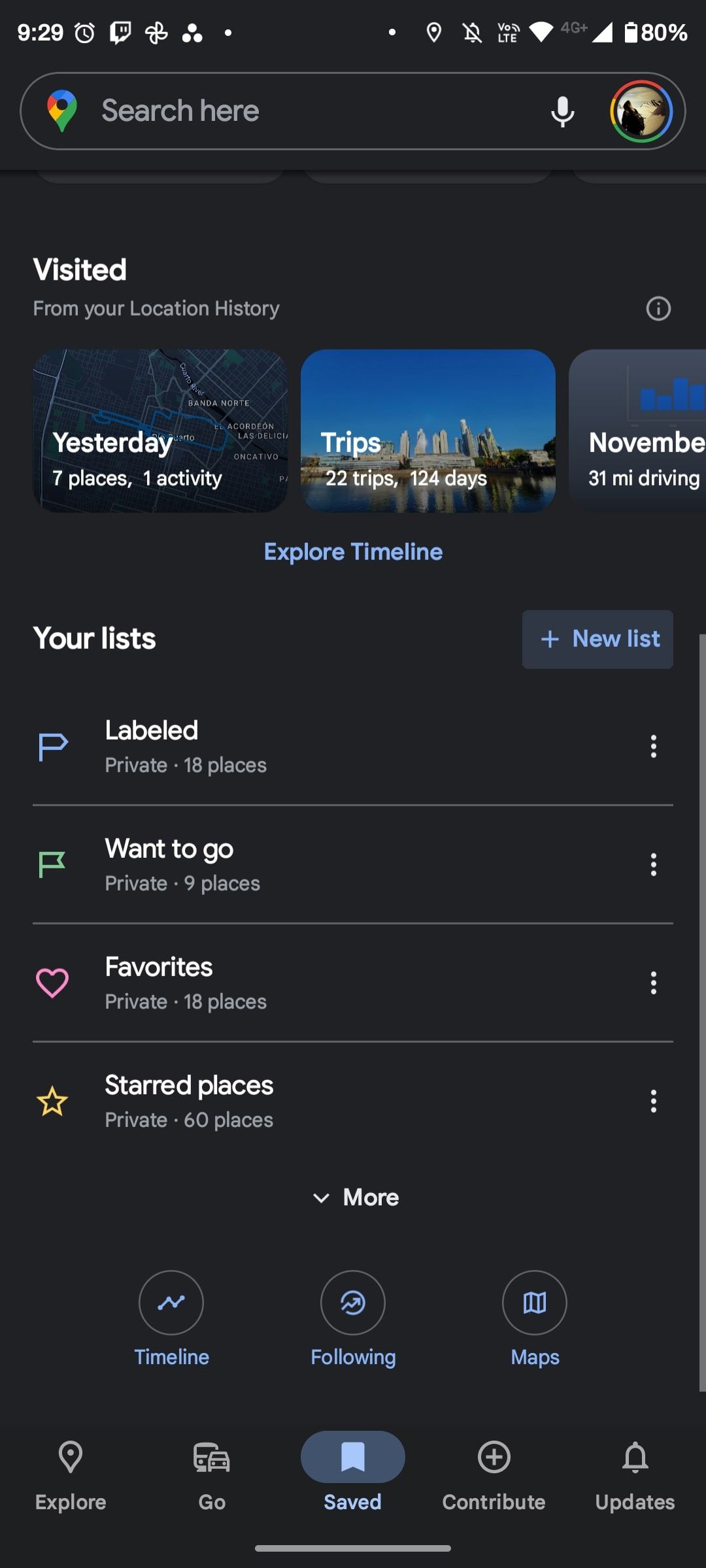This portrait-oriented cell phone screenshot, approximately three and a half times taller than it is wide, showcases various interface elements on a black background. At the very top, small white text displays standard cell phone icons. The upper left corner reads "9:29," followed by an alarm clock icon and an unfamiliar angular icon resembling a speech quote. Next, a four-petal flower icon appears alongside three white dots arranged in a pyramid, a singular white dot, and some empty black space. On the upper right, a singular white dot is followed by a location pin icon, an off-ringer bell icon, cellular strength indicator reading "LTE," and an icon representing full Wi-Fi strength. A small vertical battery bar shows 80% charge and is accompanied by the text "80%."

Below this, a search bar spans almost the entire width of the screen, with rounded corners and a black background. On its left, the Google pin drop icon appears, followed by the gray placeholder text "Search here." To the right, a white microphone icon is visible next to what seems to be a user's avatar with red, yellow, green, and blue borders.

Further down, "Visited" is prominently displayed in bold white text, left-justified. Beneath it, smaller, non-bold white text mentions "from your location history." Below these textual elements, three partially visible images are arranged horizontally. The leftmost image, a map background, is labeled "Yesterday" in white text, with "7 places, 1 activity" written beneath. The middle image shows a cityscape by the seaside, labeled "Trips" with "22 trips, 124 days" in smaller text underneath. The rightmost image, partially cut off, features blue bar charts against a gray background and reads "November" with the "R" missing, followed by "31 am I driving?" Below these images, centered in light blue text, is the phrase "Explore timeline."

Proceeding further, the section titled "Your lists" in white font introduces four rows, each featuring an icon and a corresponding label. From top to bottom, the labels are "Want to go" with a green flag icon, "Favorites" with a pink heart, "Starred places" with a yellow star, and "Labeled" with a blue flag resembling a "P." Descriptions in smaller text mark each as "private" with the number of places listed, such as "18 places" for "Labeled" and "9 places" for "Want to go." On the far right of these rows, three vertical white dots indicate additional options. Each row is separated by long light gray lines extending almost the full width of the screen.

In the bottom third of the image, the word "More" appears in white font with a downward-facing arrowhead on the left. Three blue circular icons, labeled "Timeline," "Following," and "Maps," are arranged horizontally below. At the very bottom, five equally spaced sections label "Explore," "Go," "Saved," "Contribute," and "Updates," each with corresponding icons. Notably, the "Saved" section is highlighted in blue, indicating it is selected, and features a bookmark icon.